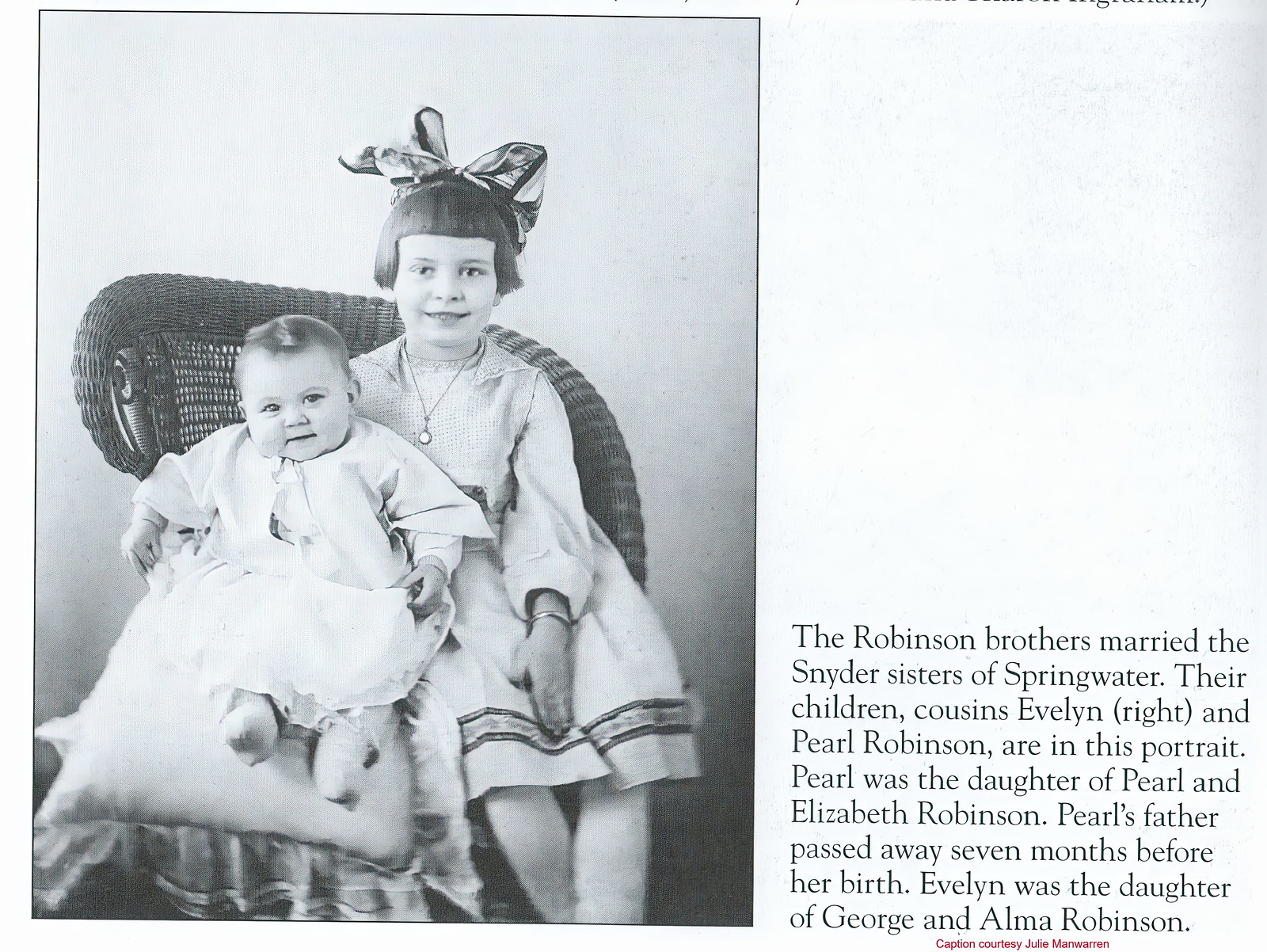This black and white portrait features two children, cousins Evelyn Wright and Pearl Robinson, seated on a woven wicker chair. Evelyn, the older of the two, appears to be around five or six years old. She wears a knee-length, long-sleeved dress, adorned with a necklace, and a large bow in her short hair. Evelyn is smiling, looking directly at the camera. On her lap, partially supported by a pillow, is baby Pearl, dressed in a long, white gown with long sleeves. The text to the right of the photograph narrates their family history: "The Robinson brothers married the Snyder sisters of Springwater. Their children, cousins Evelyn Wright and Pearl Robinson, are in this portrait. Pearl was the daughter of Pearl and Elizabeth Robinson; her father passed away seven months before her birth. Evelyn was the daughter of George and Alma Robinson." The image captures a moment of familial bond, set against a timeless monochrome background.